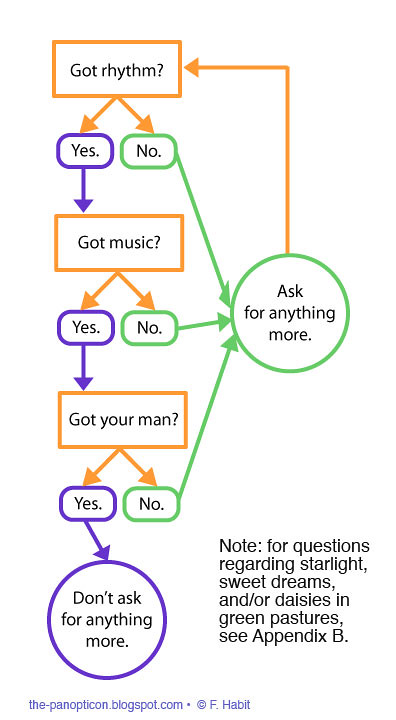The image is an informational diagram in portrait orientation, featuring a clear, color-coded flowchart with branches and labels in orange, green, and purple. The diagram begins in the top section with three main questions in orange boxes: "Got rhythm?" followed by "Got music?" and "Got your man?" Each question presents a binary choice with options "yes" or "no." If "yes" is selected, the flow continues to the next question, while a "no" leads to a green box stating, "ask for anything more." The sequence culminates in the bottom with a purple circle reading "don't ask for anything more" if all are "yes." 

The bottom right of the diagram includes additional instructions in black text for further inquiries related to "starlight, sweet dreams, and/or daisies in green pastures," directing the viewer to "see Appendix B." In the very fine print at the bottom left, attributed to "thepanopticonblogspot.com, copyright F habit," the diagram emphasizes a whimsical, detailed navigation through a set of conditions and outcomes.